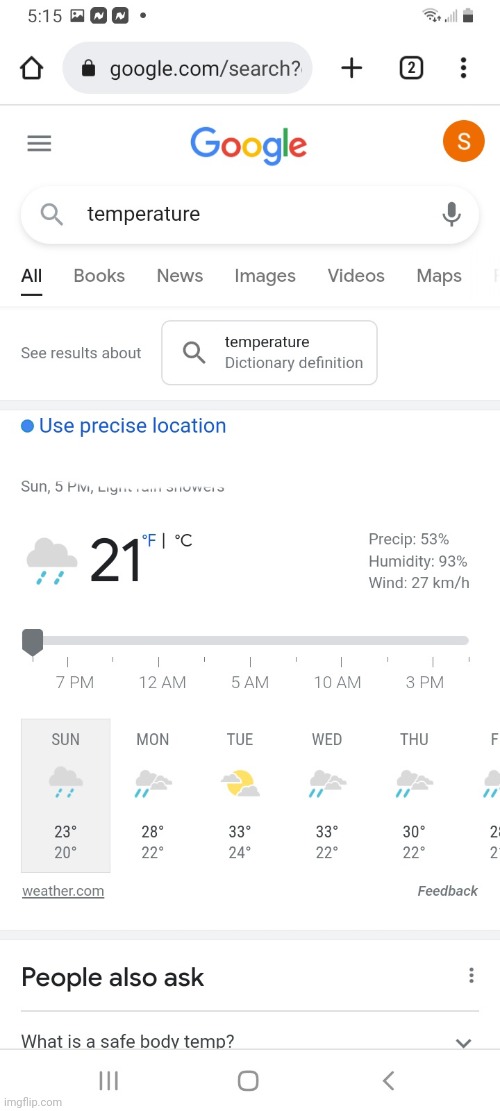The image appears to be a screenshot from a smartphone displaying a Google search result about the current weather. The background is white with black text. Situated at the top left is the time, reading 5:15. On the far right, there are icons for Wi-Fi, battery, and network signal, the last of which has only one filled bar. Below these, there is a home icon and a search bar or website bar, indicating the user is on Google. 

Underneath, the word "Google" is visible, with an orange circle and the letter "S" to its right. Below this logo, there is a search bar containing the word "temperature." To the left of "temperature" is a search icon, and to the right is a microphone icon. 

Further down, a set of filter options is displayed, listing "All, Books, News, Images, Videos, Maps." Below this, a subheading "See results about" introduces the box displaying the "temperature dictionary definition." It's followed by a hyperlink in blue reading "Use precise location."

Subsequently, a weather summary shows a cloud icon with rain, a current temperature of 21 degrees Celsius, 53% precipitation, 93% humidity, and a wind speed of 27 kilometers per hour. 

A gray box underneath shows a weather forecast for Sunday, marked by rain with temperatures ranging between a high of 23 degrees and a low of 20 degrees.

At the bottom of the screen, a section titled "People also ask" is visible, listing the query "What is a safe body temperature?"